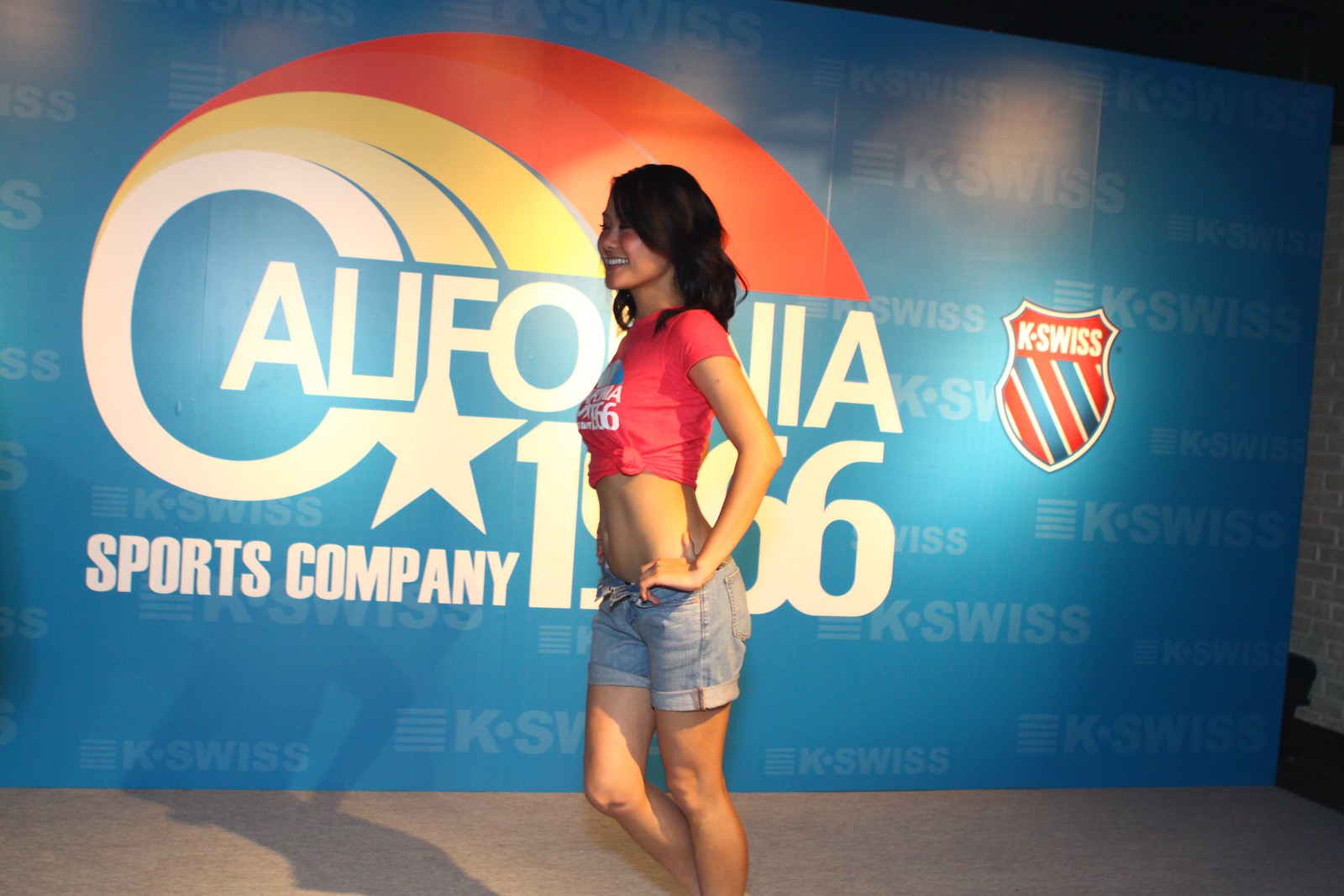In this image, we see a young woman standing indoors in front of a large, rectangular banner that reads "California 1966 Sports Company" and features the K-Swiss logo. The banner is predominantly light blue with "California 1966 Sports Company" written in white text. Surrounding the word "California" is a stylized semi-circle resembling a rainbow, composed of white, light yellow, deep yellow, light red, and deep red colors. The K-Swiss shield logo, situated towards the top right of the banner, includes red and blue stripes with white text.

The woman, who is dark-haired with wavy locks and light skin, is positioned centrally in the image and is turned slightly to the side, facing left. She is smiling, adding a cheerful element to the scene. Her outfit consists of a tied-up red crop top that also says "California 1966" in white lettering, similar to the banner, and light blue jean shorts. The setting resembles an event or an award ceremony, suggested by the indoor stage-like gray surface at the bottom of the image. Various colors in the image include black, blue, orange, yellow, white, light blue, red, tan, and gray, contributing to a vibrant and dynamic atmosphere.